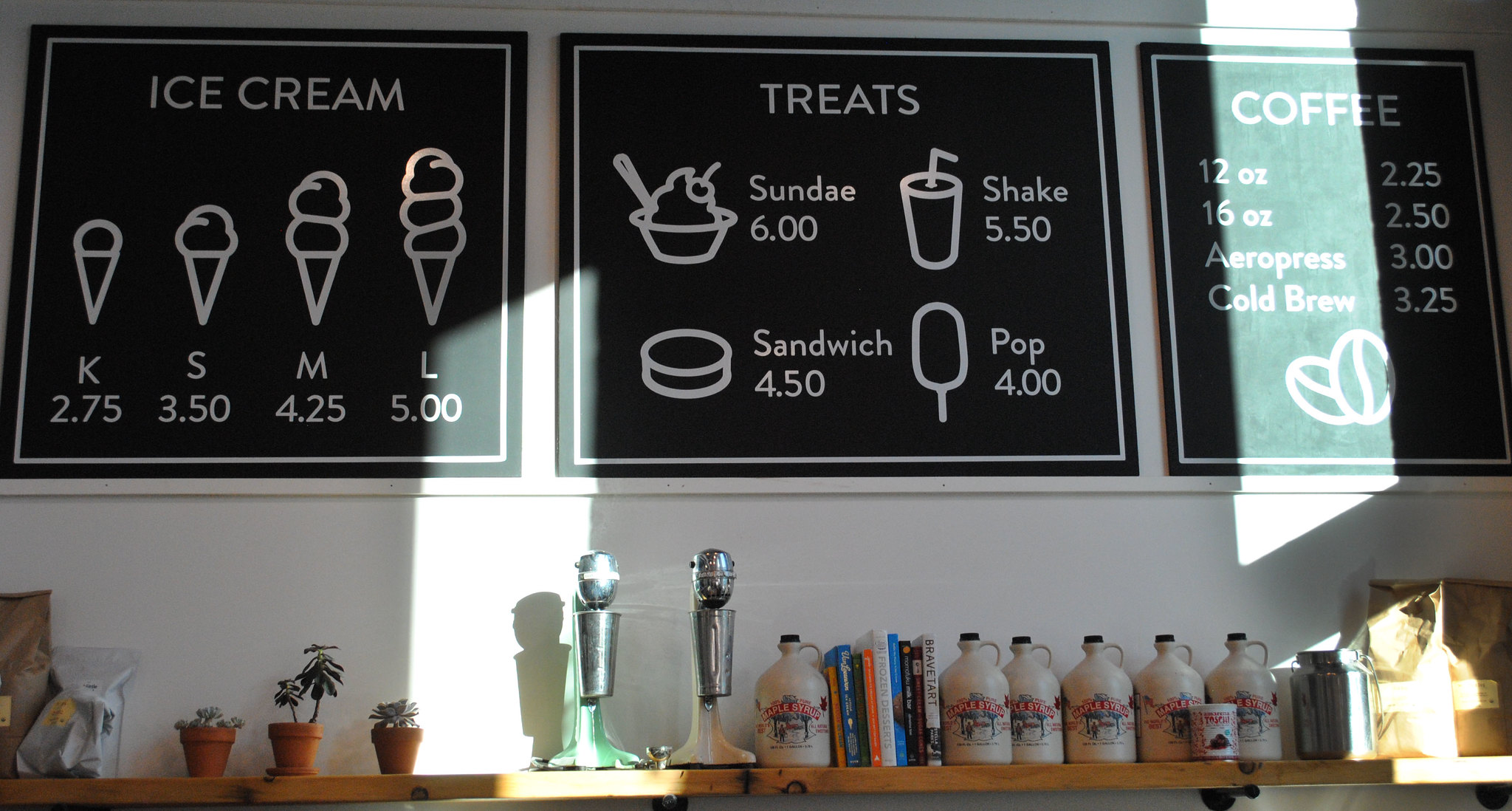This image is a detailed, color indoor photograph capturing the back of an ice cream parlor, focusing on three black signs with white text and drawings, mounted above a rustic wooden shelf filled with various items. 

The leftmost sign features a small white box border and reads "ICE CREAM" in capital letters at the top. Beneath this, drawings illustrate different ice cream cones labeled with letters and prices: "K" for a single small scoop at $2.75, "S" for a slightly larger single scoop at $3.50, "M" for two scoops at $4.25, and "L" for three scoops at $5.00.

The middle sign is titled "TREATS" and features illustrations of various desserts along with their prices: a sundae for $6.00, a shake for $5.50, an ice cream sandwich for $4.50, and a pop for $4.00.

The rightmost sign lists coffee options with accompanying prices and includes a small drawing of coffee beans: a 12-ounce coffee for $2.25, a 16-ounce coffee for $2.50, AeroPress coffee for $3.00, and cold brew for $3.25.

Below these signs, a wooden shelf holds an array of items. From left to right, the shelf displays some bags, three small ceramic plant pots, two upright milkshake mixers with silver cups attached, several upright gray jugs of syrup, some books sandwiched between the jugs, and more bags and containers on the right. The wall behind the shelf is white, providing a bright backdrop that highlights the shop's assortment.